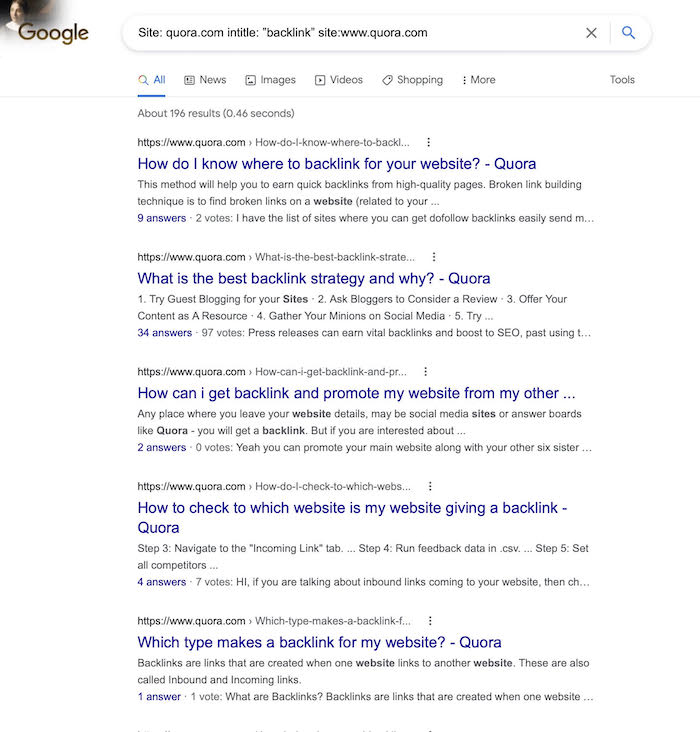A Google search results page is displayed with a brown Google logo in the upper left-hand corner. In the search bar, the query entered is "site:quora.com backlink site:www.quora.com." 

The page prominently features an image of a nun looking to the side. Below the search bar, a series of search results from Quora are listed, each with clickable blue links underlined for emphasis.

1. The first result is titled, "How do I know where the backlink for your website? Where to backlink for your website Quora."
2. The second result is titled, "What is the best backlink strategy? Why?" This entry shows it has 97 upvotes.
3. The third result down is titled, "How can I backlink and promote my website from my other," though the title is cut off.
4. Further down, another result reads, "How to check to which website is my website giving a backlink."
5. The final visible result asks, "Which type makes a backlink for my website."

All results are from Quora, showing various responses and a count of upvotes ranging from 1 to 97. Additional answer counts are visible, indicating community interaction.

Above the search results, options such as "All," "News," "Images," "Videos," "Shopping," "More," and "Tools" can be seen, offering filtering options for the search results.